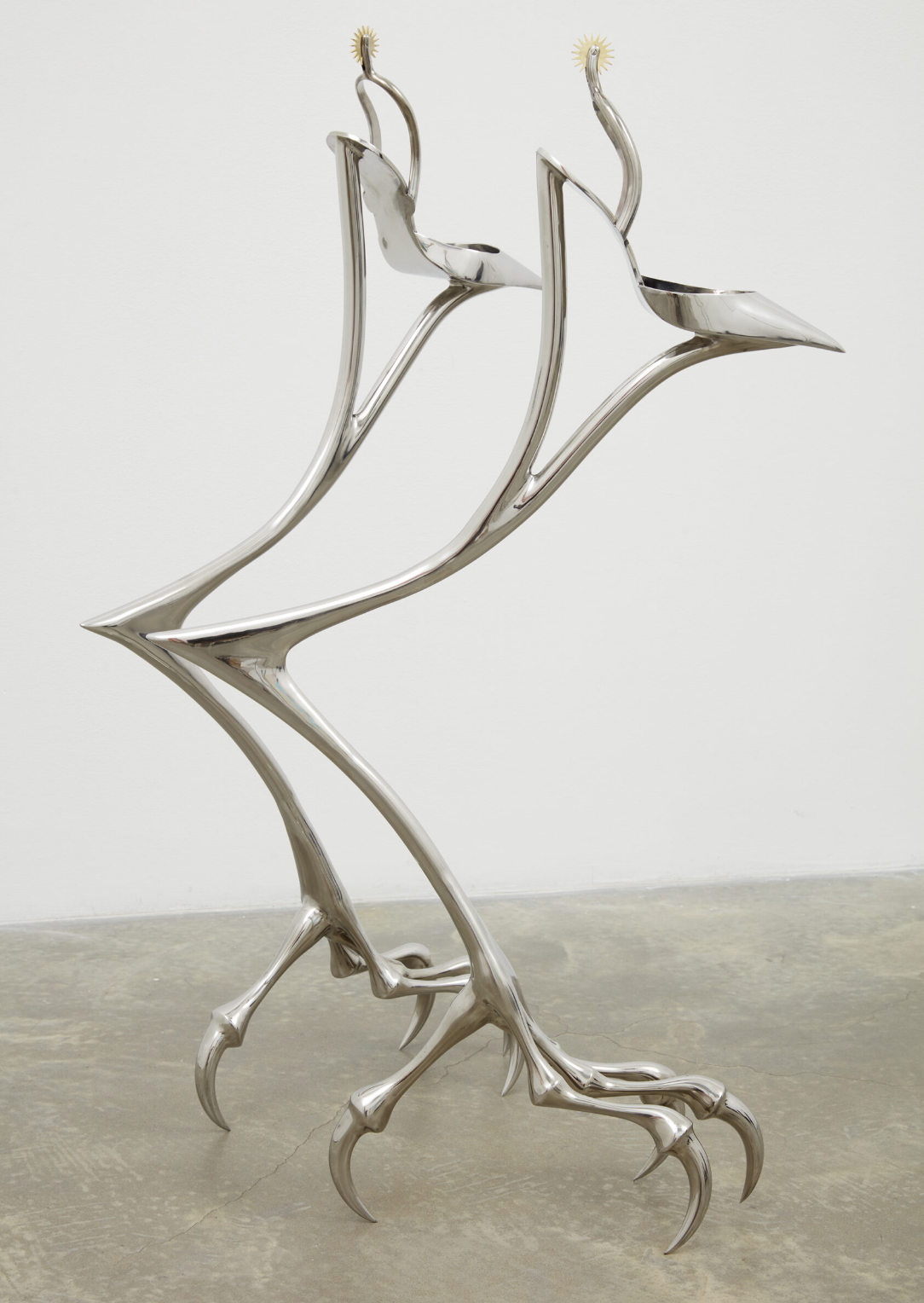This photograph features a striking modern art sculpture set against an off-white painted wall and resting on a gray cement or marble-like floor. The sculpture is crafted from silver metal and intricately designed to resemble a pair of high-heeled shoes morphing into realistic bird legs. Each shoe's heel elongates into an elegant, stylized bird leg, complete with detailed talons resembling those of a predatory bird like an eagle or falcon. The ankles have a lifelike bend and form, contributing to the lifelike illusion before becoming more abstract. Where a foot would rest in the high heel, the metallic structures culminate in ornate yellow spurs, adding a unique and dynamic twist to the piece. This dual structure stands tall with three talons placed forward and one extending back, giving a balanced, yet commanding presence that blurs the line between fashion and nature-inspired fantasy.